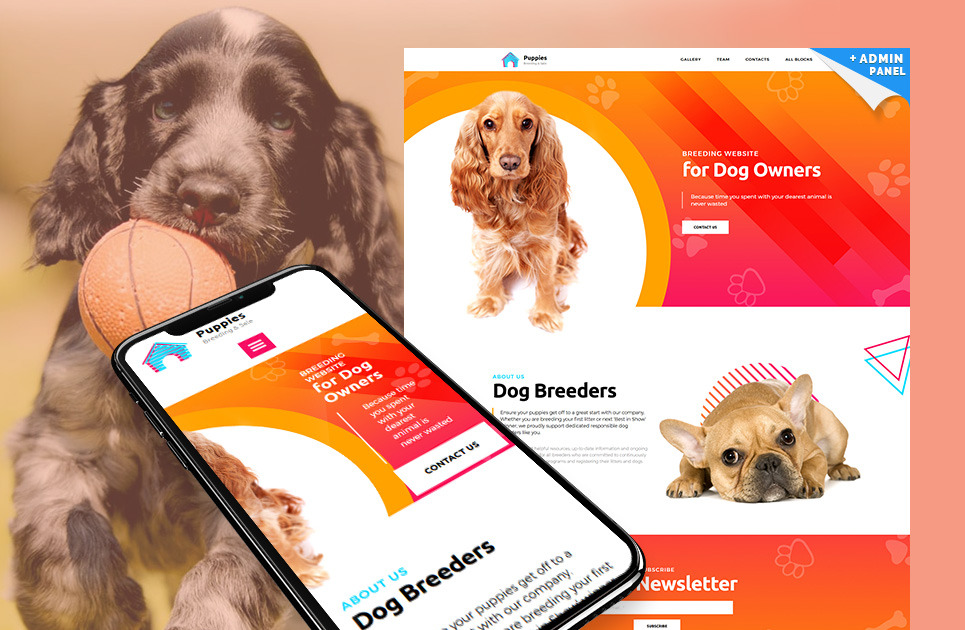This advertisement graphic is designed for dog enthusiasts, particularly targeting dog owners and potential dog breeders. 

The left side of the image prominently features a young Spaniel with medium-length, dark gray fur that has lighter gray and white patches. The dog's striking bright blue eyes and a basketball-colored ball held in its mouth make it an endearing focal point.

On the right side, the image showcases the homepage of a website being advertised. The webpage design incorporates a vibrant orange and red background, divided into sections with a prominent white area in the center and to the left. This layout is mirrored on a smartphone graphic, suggesting that the site is compatible with mobile devices. 

Additionally, there are a couple of other dog images featured on this side. One is a golden-colored Spaniel with light fur, and another is a tan-colored French Bulldog. The graphic prominently displays black text reading “Advertising Dog Breeders,” followed by a smaller, medium gray description underneath. 

This detailed composition effectively communicates the purpose and design of the advertisement, appealing to dog lovers and those interested in dog breeding.